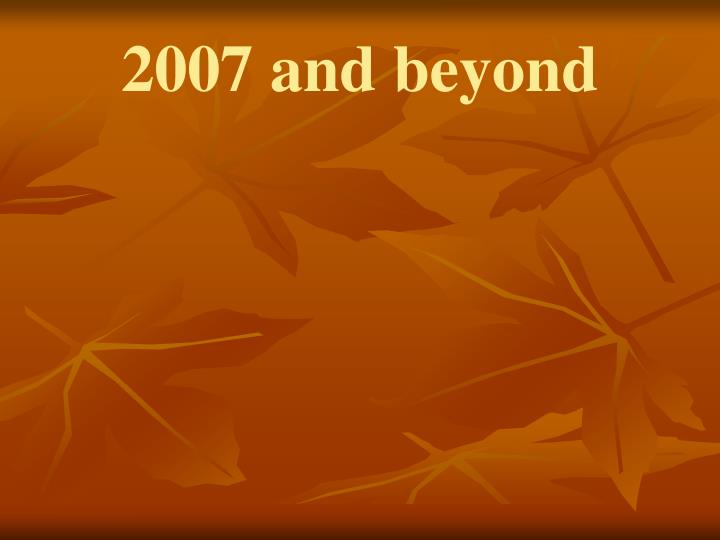The image features a square patterned background dominated by various shades of orange. It includes a detailed leaf motif where the leaves are illustrated in both lighter and darker hues of orange, enhancing their visibility against the more subdued backdrop. The top of the image displays the text "2007 and beyond" in white letters, centered and prominent under a darker shadowed area. The leaves are arranged in a scattered yet deliberate manner, with some pointing left and right, and others facing downward. The upper portion has a leaf sticking out and another pointed towards the right, while the lower part includes a leaf at the bottom left corner pointing downward and another on the right side pointing left. A gradual gradient border at the top and bottom of the image transitions to a darker shade, creating a shadow effect that frames the design. The overall feel is suggestive of a fall theme, encapsulated by the warm, autumnal palette and leaf imagery.